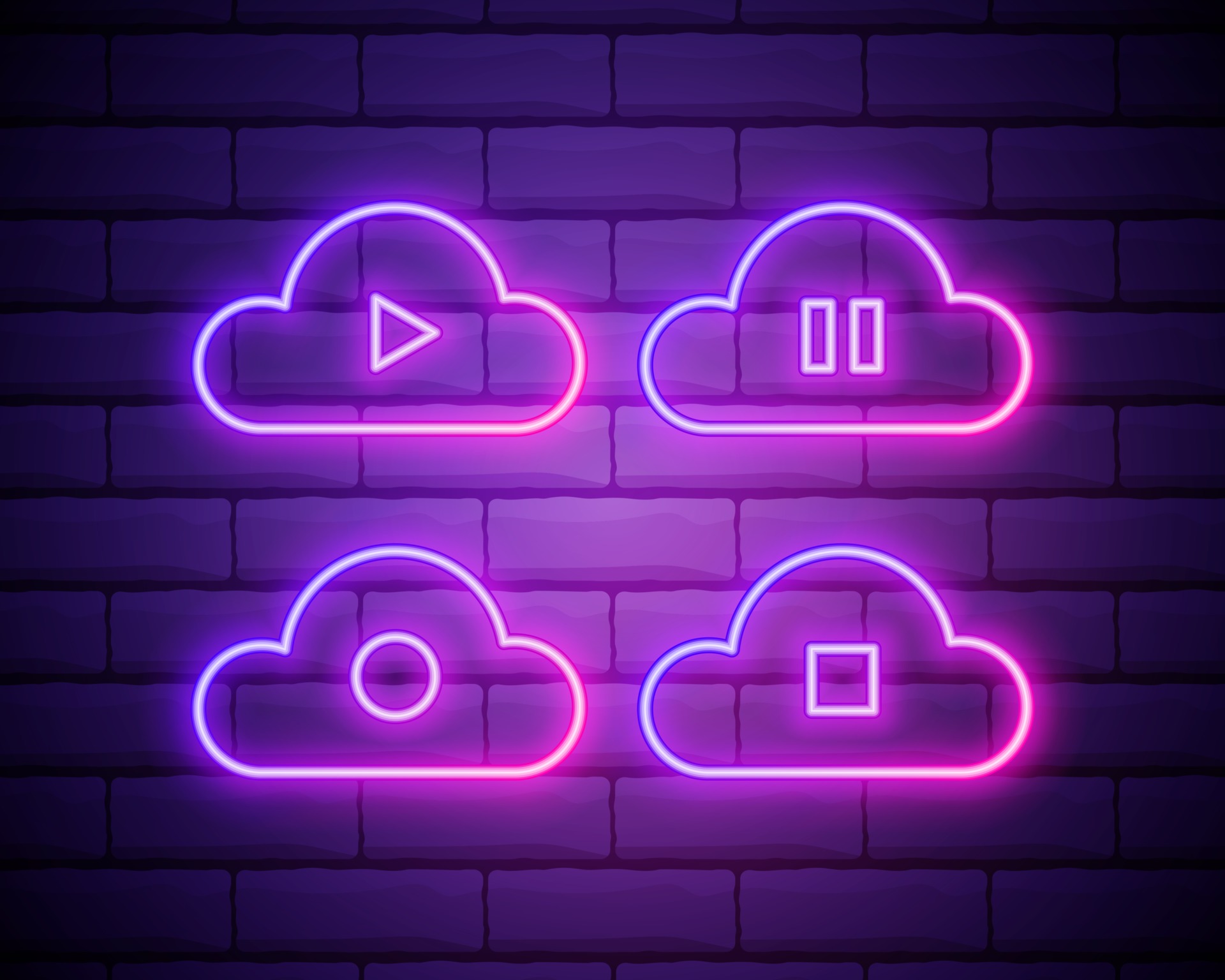This vibrant rectangular digital artwork features an abstract depiction of a brick wall with a striking purple hue. The background showcases horizontally aligned, overlapping bricks, accentuated by black grout lines and a prominent black vignette that fades toward the center, creating an ombre effect from dark black at the corners to a lighter purple at the middle. Embedded on this wall are four glowing, cloud-shaped neon lights, each exuding a mesmerizing blend of pink, purple, and hints of blue. These neon clouds, evenly spaced with two at the top and two at the bottom, each contain a distinctive symbol: a triangle in the top left cloud, two vertical bars in the top right, a circle in the bottom left, and a square in the bottom right. The glowing icons within these neon clouds create a dynamic, luminous focal point against the animated purple-black brick background, evoking a sense of digital futurism.